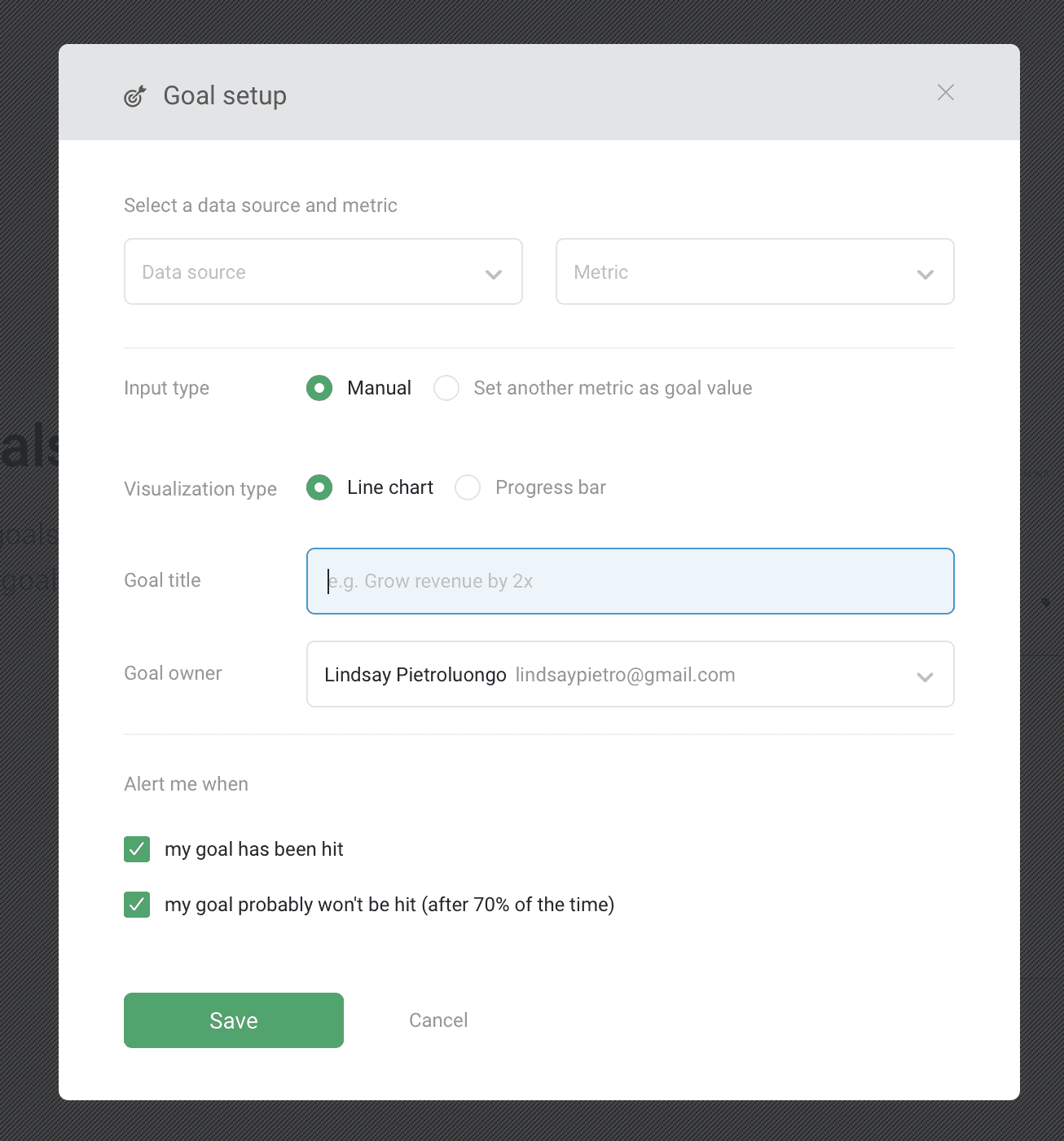The image is an interface screen with a black border. At the top, a blue box with a target and arrow icon displays the text "Goal Set Up," with an "X" button on the right side for closing the window. Below this is a large white section that prompts users to "Select the Data Source and Metric."

In this section, there is a dropdown box labeled "Data Source" and another dropdown labeled "Metric." Further down, the "Input Type" area features a green circle with a white center labeled "Manual." There is also an option to set another metric for "Goal Value."

Next is the "Visualization Type" section, which includes options for displaying the data via a line chart or a progress bar, each indicated by a green circle with a white center.

The "Goal Title" field is presented in a blue box with the placeholder text "Grow Revenue by 2X." Below this, the "Goal Owner" section includes a box with the name "Lindsay Pietralongo" and her Gmail address. There's also a dropdown arrow for selecting different owners.

The "Alert Me When" section follows, showing two green boxes with check marks. The first box specifies "My Goal Has Been Hit," and the second states "My Goal Probably Won't Be Hit After 70% of the Time."

At the bottom of the interface, there is a large green "Save" button alongside a white "Cancel" button.